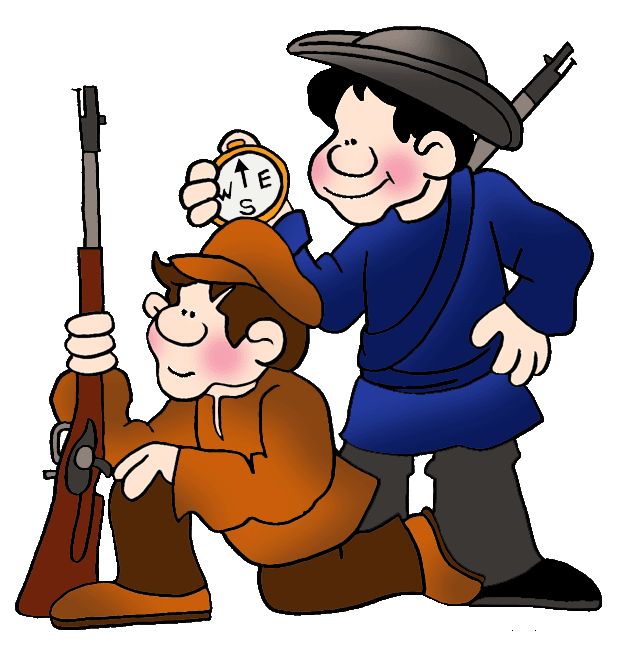The image is a cartoonish comic book-style illustration of two white, rosy-cheeked male hunters on a white background. The hunter on the left is kneeling with a slight smile, wearing brown pants, an orange-brown shirt, and a matching brown train-style cap that covers his brown hair. He holds a musket or shotgun with three fingers of his right hand, pointing it upward, while his left hand is rested on his knee. The second hunter stands behind him, wearing a blue tunic, gray pants, and brown shoes. He has a dark gray fedora-like hat atop his brown hair and is smiling while holding a compass in his right hand, which is pointing north. His left hand is on his hip, and a musket or shotgun is strapped across his back. Both hunters have simplified features, including large noses and three fingers and a thumb on each hand, giving them a distinct cartoonish appearance. They both seem to be looking off into the distance.